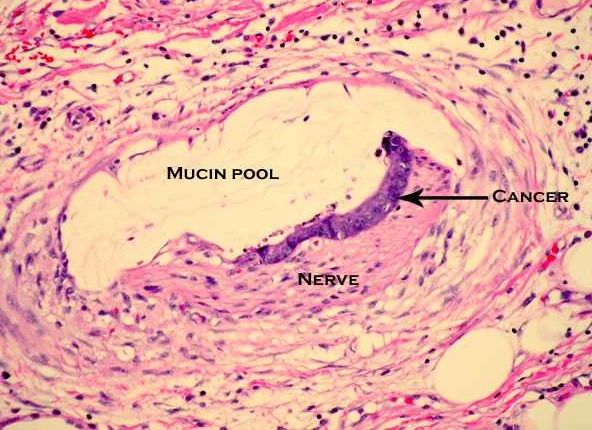The image appears to be a detailed, color-enhanced photograph taken through a microscope, showcasing a microscopic view of cancer cells. Central to the image is an off-white, oval-shaped area labeled "mucin pool" in black text, resembling a pool. Surrounding this mucin pool are interlacing pink and purple cell walls, with dark purple sections outlining its perimeter. To the bottom right of the pool, the term "cancer" is labeled in black text, accompanied by a leftward-pointing black arrow indicating the dark purple perimeter where the cancer cells are likely concentrated. Below and to the left of this area, another black label reads "nerve," indicating the proximity of the nerve tissue to the cancerous region. Additional visual elements include various black dots and purple swirls throughout the image, further detailing the cellular structures.